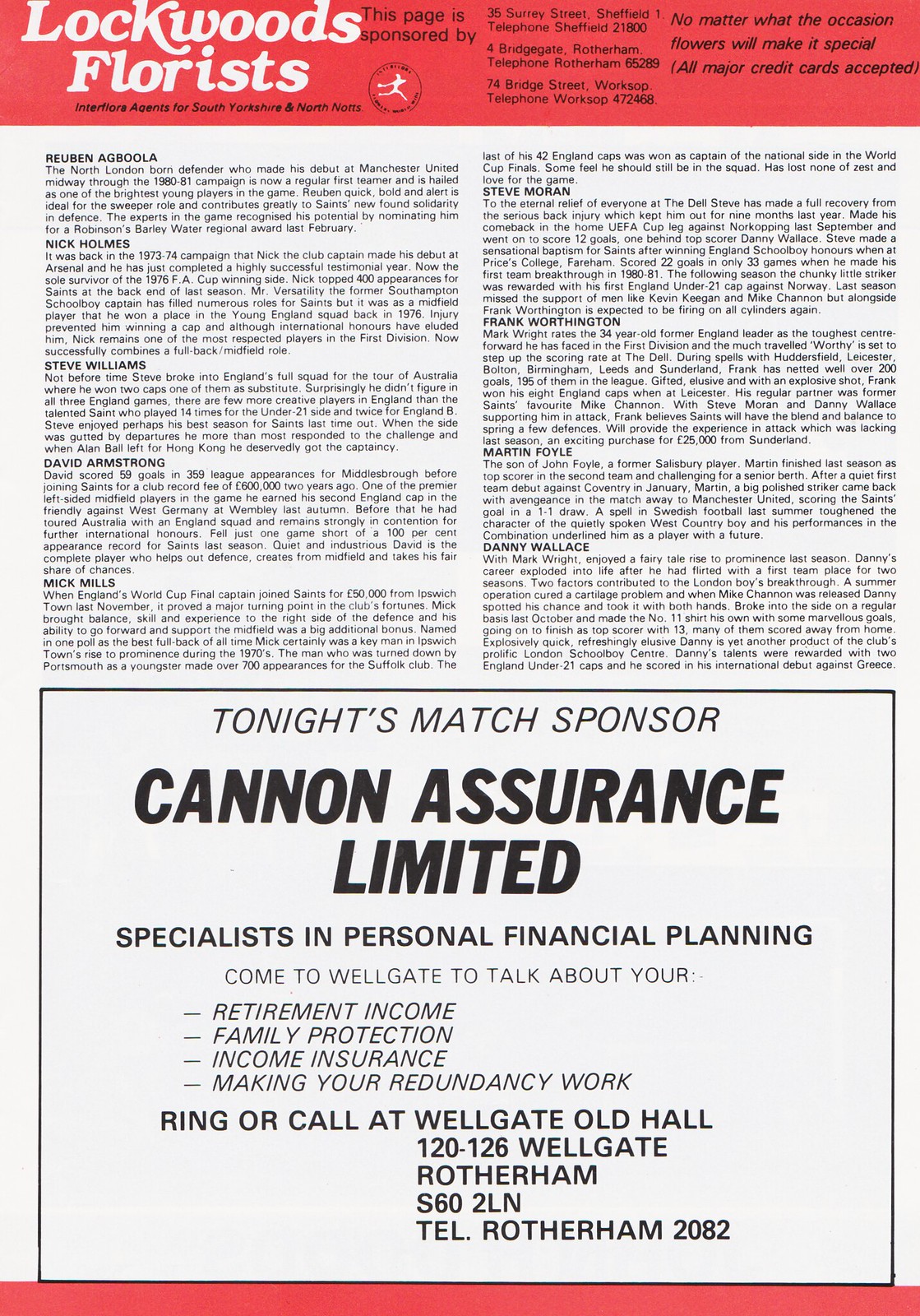This flyer is an intricate promotional piece for Lockwood's Florists, an Interflora agent serving South Yorkshire and North Nottinghamshire in the UK. At the very top, a striking red banner prominently displays the sponsorship details, including addresses and phone numbers for three locations: 35 Surry Street, Sheffield (Telephone: Sheffield 21800), 4 Bridgegate, Rotherham (Telephone: Rotherham 65289), and 74 Bridge Street, Workshops (Telephone: Workshop 472468). The banner also features the tagline "No matter what the occasion, flowers will make it special," along with a note that all major credit cards are accepted. 

Centrally, the flyer showcases a detailed article focused on Reuben Agboola, the North London-born defender who debuted with Manchester United midway through the 1980-81 season. Now a regular first-team player, Agboola is praised as one of the brightest young players in football, being ideal for the sweeper role and enhancing Saints' defense. His potential has been recognized by being nominated for a Robinson's Barley Water Regional Award last February. 

Additionally, the flyer lists names and descriptions of other athletes, highlighting their careers and contributions, though the print is notably small. 

At the bottom, another advertisement introduces tonight's match sponsor, Canon Assurance Limited, specialists in personal financial planning. This section outlines their services, including retirement income, family protection, and income insurance, along with their business address and contact information. This meticulously crafted flyer combines multiple promotional elements aimed at engaging a diverse audience.